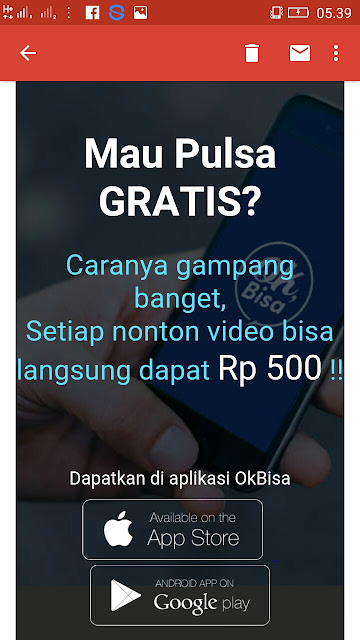The image appears to be a screenshot of a mobile app promotional page. At the very top, there's a dark red horizontal bar featuring the Facebook logo, the time "5:39," a signal indicator, and a half-charged battery icon. Below this bar, there are white symbols: a left-facing arrow, a recycling bin, a mail envelope, and a vertical ellipsis (three dots).

Beneath this top bar, the central section of the image showcases a partially visible hand holding a smartphone with a blue screen. The screen displays a white circle with the word "Visa" inside it.

Overlaying this background image, in the upper part, is text in white that says "Mau Pulsa Gratis?" Below that, blue and white text states "Karena Gampang Banget, Setiap Nonton Video Bisa Langsung Dapat RP 500!!" In a few lines of white text underneath, there are the letters "D-A-P-A-T-K-A-N D-I A-P-L-I-K-A-S-I O-K B-I-S-A."

At the bottom of the image, there are buttons for downloading the app, highlighted in white. One button reads "Available on the Apple Store" with the Apple logo next to it, and another button states "Available on Google Play" with the Play Store icon beside it.